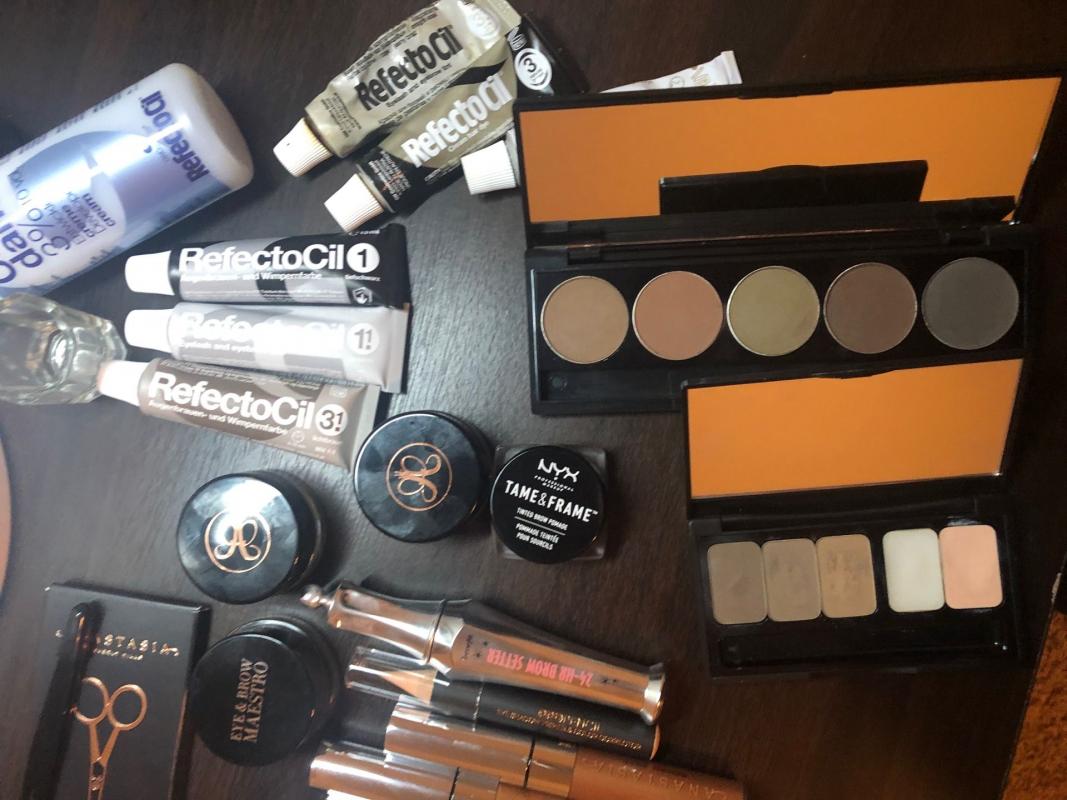The image depicts a dark black wooden tabletop with makeup items scattered across it. Dominating the scene is a palette featuring various eyeshadow shades, including brown, reddish-brown, green, dark red, blue, and orange, arranged in square compartments alongside white and pink hues. 

In the top left corner, there are several items including a bottle and two tubes labeled "RefectoCil." Additionally, there are three tubes positioned towards the left side, also labeled "RefectoCil," in black, silver, and gray colors. 

On the bottom left, there is a black jar adorned with a small butterfly symbol. Further to the right, another black jar is visible with white text that reads "NYX Tame and Frame." Among these items, there is also a black jar featuring a scissors symbol, and a collection of various tubes scattered around the tabletop.